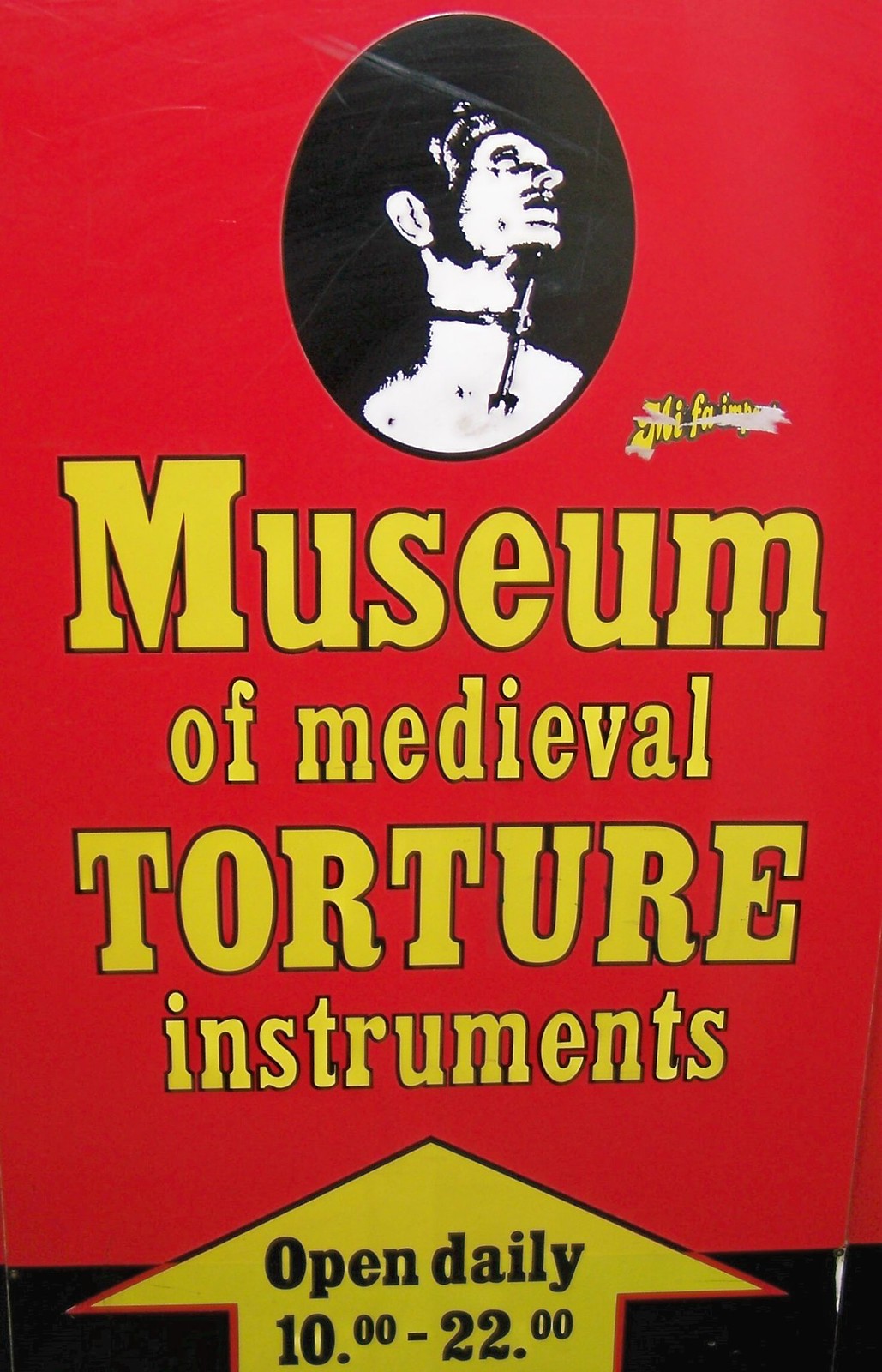This is a vividly detailed poster advertisement for the Museum of Medieval Torture Instruments. The background is a rich red, dominated at the top by a black circle containing a black-and-white sketch of a person's head wearing what appears to be a medieval torture device around their neck. The bold, yellow text in the center of the poster announces "Museum of Medieval Torture Instruments." Below, a yellow arrow outlined in black and red points upward with the text "Open Daily, $10 to $22" in black font. To the right of the circular image at the top, there is an unreadable yellow inscription, possibly a signature. The color scheme of the poster is mainly red, yellow, black, and white, emphasizing the stark contrast and drawing the viewer's focus to the critical details of the advertisement.